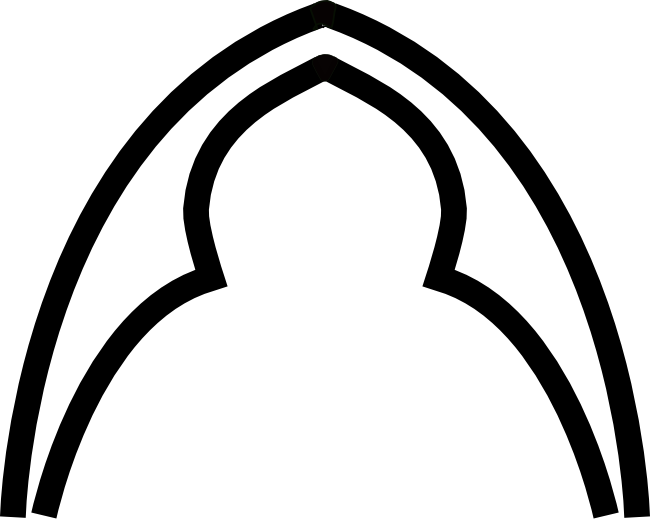The image is a minimalist black-and-white drawing on a white background, featuring two sets of thick black lines that form arch-like structures. The outer set consists of two curved lines, resembling an elongated oval with pointed ends, similar to the outline of a bishop's hat in chess or a keyhole's top half. Within this outer structure, there is a similar but smaller set of lines on each side, creating a tunnel-like appearance. The inner lines, also curved with pointed ends, further emphasize the archway effect, akin to a wedding arch or a decorative doorway. The drawing's simplicity is underscored by its stark contrast and minimal detailing.